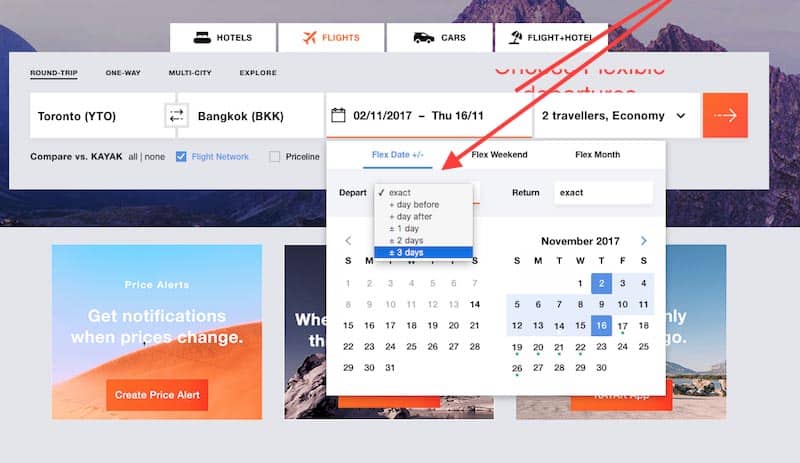The image is an instructional infographic from a travel website, providing users with detailed navigation for booking flights. At the top of the infographic, there are navigation tabs labeled "Hotels," "Flights," "Cars," and "Flight + Hotel." The "Flights" tab is currently selected. Below this, users can choose between different trip types with buttons for "Round Trip," "One-Way," and "Multi-City Explorer," with "Round Trip" being the selected option.

The flight details section indicates a journey from Toronto (YTO) to Bangkok (BKK), scheduled to depart on November 2, 2017, and return on Thursday, November 16, 2017. The booking involves two traveler tickets in the Economy class. A large right arrow button suggests proceeding to the next step in the booking process, and users have the option to compare prices with Kayak via the comparison tool below.

There is also a "Flight Network" button, though its function is not entirely clear from the image, and an unselected "Priceline" button. The lower part of the box is partially obscured by a date selection calendar, which displays the November 2017 calendar with the 2nd and 16th highlighted.

An arrow points to a "Flex Date" box, which allows for date flexibility by plus or minus 3 days. At the bottom right, there is a "Price Alerts" feature, encouraging users to get notifications when prices change. Additionally, there are two partially covered buttons that depict different landscapes: one shows a desert background, and the other two, possibly, mountains.

This detailed, step-by-step visual guide assists users in navigating their flight booking process, ensuring clarity and ease of use.